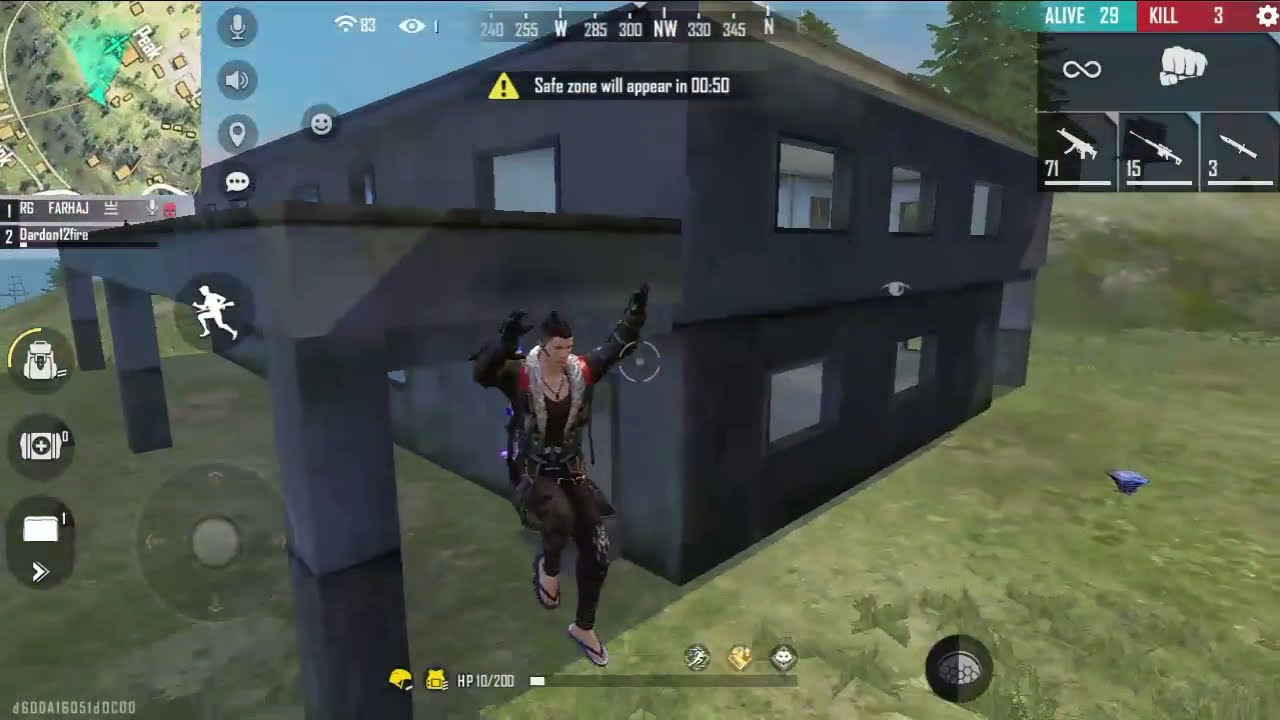This screenshot captures a dynamic scene from a battle royale video game, likely PUBG or Free Fire. Dominating the center is a two-story, gray stucco building with an overhang and multiple windows. A male character is mid-air, having apparently jumped from the building's overhang. He is clad in a black jacket, black tank top, black parachute pants, and dark flip-flops. His accessories include black gloves and a headset with an earpiece and microphone, with his hair tied in a bun.

To the left of the building, the ground is carpeted in green grass, which also extends to the foreground and right side of the image. In the upper left corner, a map is visible, along with a compass strip that reads "255 W 285 300 NW 330 3 4 5 North," and features a gold triangle with an exclamation point, indicating "Safe zone will appear in 0:50."

In the upper right corner, there are icons for various weapons, which include a rifle, a knife, and a fist, along with game stats showing "Alive: 29" and "Kills: 3." The bottom middle of the screen displays an HP icon. A serene water body can be seen in the upper left corner of the image, adding contrast to the intense action taking place.